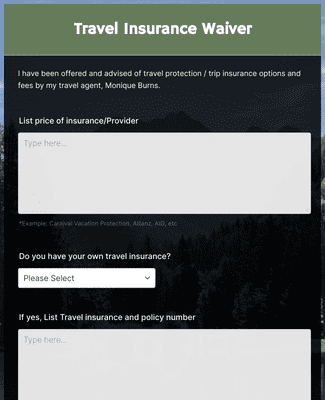Screenshot of a smartphone displaying a travel booking interface, specifically a pop-up window for a travel insurance waiver. The top of the pop-up features a light olive-green field with centered white text. Below this, there's an overlay that partially covers an image of pine trees on a mountain background, visible through the edges. 

The main text reads: "I have been offered and advised of travel protection/trip insurance options and fees by my travel agent, Monique Burns." Below this, there's a white input field labeled "List price of insurance provider" with a placeholder text "Type here...".

An example is provided underneath, though partially obscured, possibly reading "Carnival Vacation Protection". Further down, a drop-down menu labeled "Do you have your own travel insurance?" prompts the user to make a selection. If "Yes" is selected, additional fields appear for entering the travel insurance provider and policy number.

The pop-up aims to confirm whether the user wants to waive the offered travel insurance, either because they have their own or prefer to pay for the offered insurance, which can affect the overall booking price.